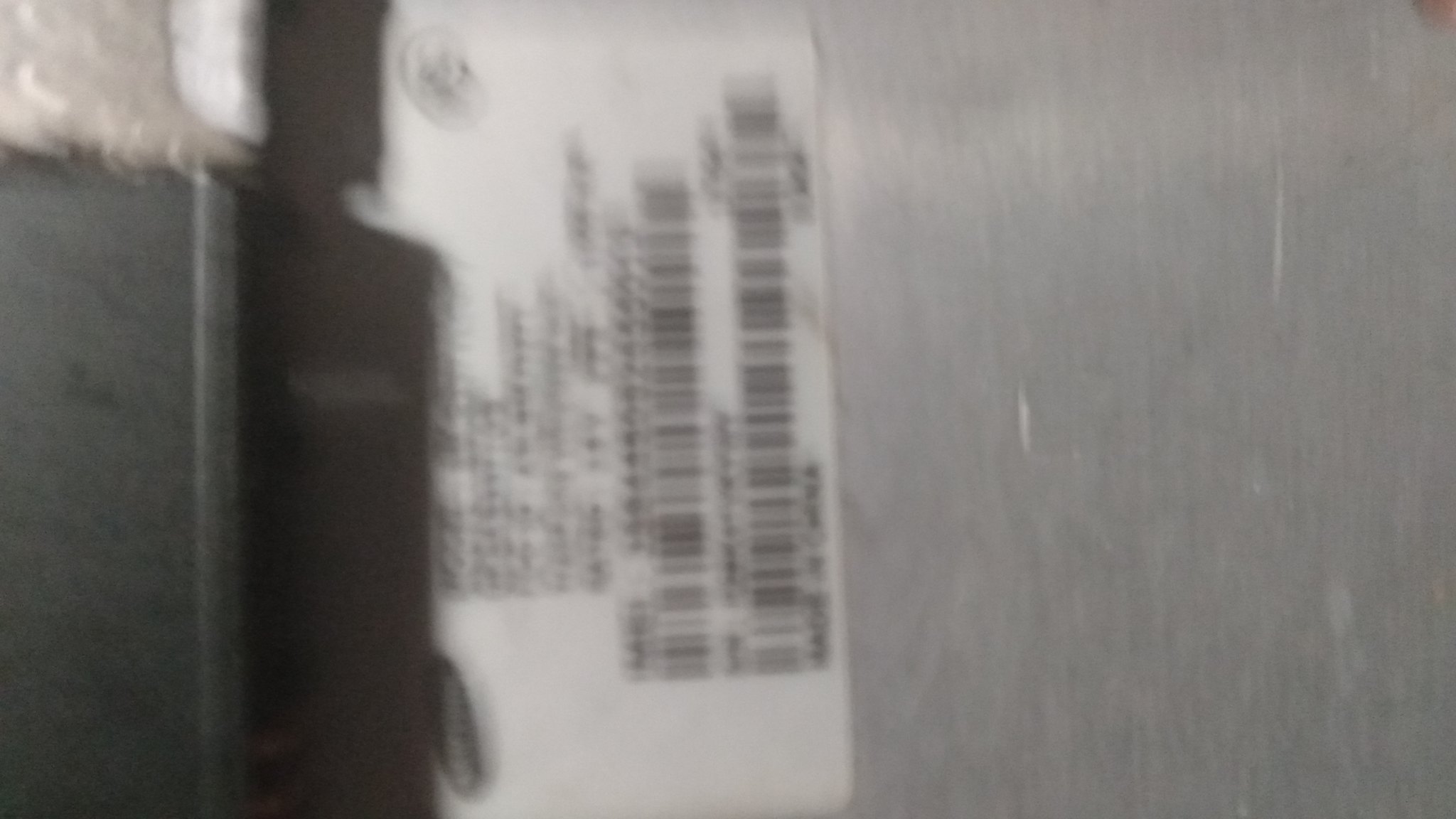This image captures a severely blurred photograph, likely taken overhead in poor lighting conditions, showcasing the back of an electronic device, possibly a cellphone or a laptop. The device appears to be grey or silver in color, with a black rectangular section and an elevated border casting a shadow. Prominently featured is a white label containing multiple barcodes and text, including what seems to be an IMEI number and potentially the Samsung logo, situated in the top left corner of the label. The overall lack of focus makes it difficult to discern specific details, suggesting movement during the photograph's capture or failure to focus properly. The label resembles those used for company-issued devices, displaying critical device information despite the image's indistinctness.